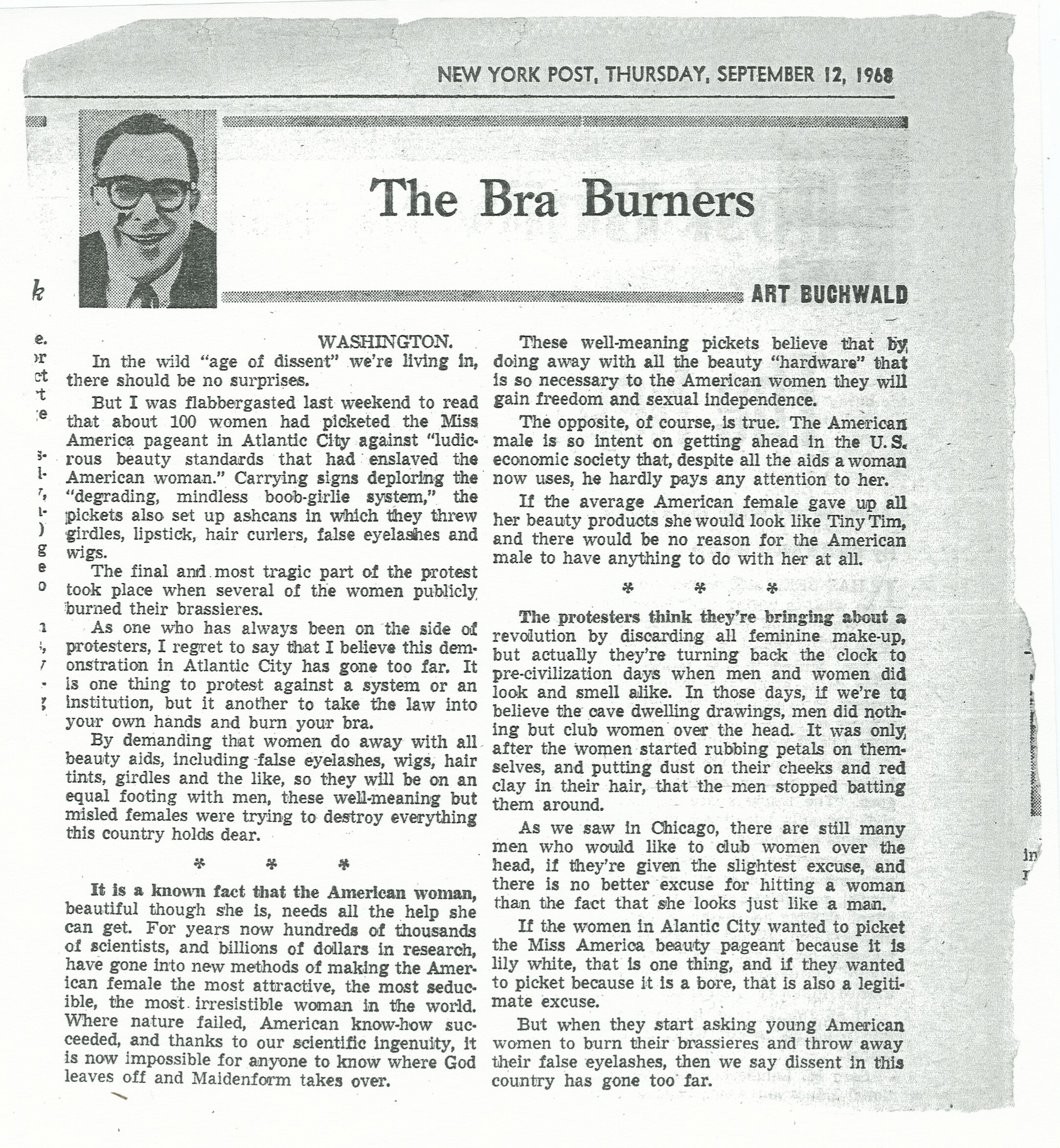This is a scan of a newspaper article from the New York Post dated Thursday, September 12, 1968. The newspaper's name and the date are prominently printed in black ink in the upper right corner. The article, titled "The Bra Burners," is authored by Arch Buchwald, whose black-and-white portrait appears on the top left corner. The image shows that the newspaper edges are torn and uneven, enhancing its aged appearance. The headline "The Bra Burners" is centered and bold. The article details an event where approximately a hundred women protested against restrictive beauty standards by targeting the Miss America pageant in Atlantic City. These demonstrators expressed their dissent by burning bras and other beauty aids such as wigs and makeup, aiming to challenge and spotlight the oppressive norms imposed on women. The language used in the article is noticeably outdated and sexist, reflecting the era's societal attitudes. The content begins with the line, "Washington, in the wild age of dissent we're living in, there should be no surprises. But I was flabbergasted last weekend to read about a hundred women that had picketed the Miss America pageant in Atlantic City against ludicrous beauty standards that had enslaved American women," and continues in a similar vein throughout several paragraphs on the page.